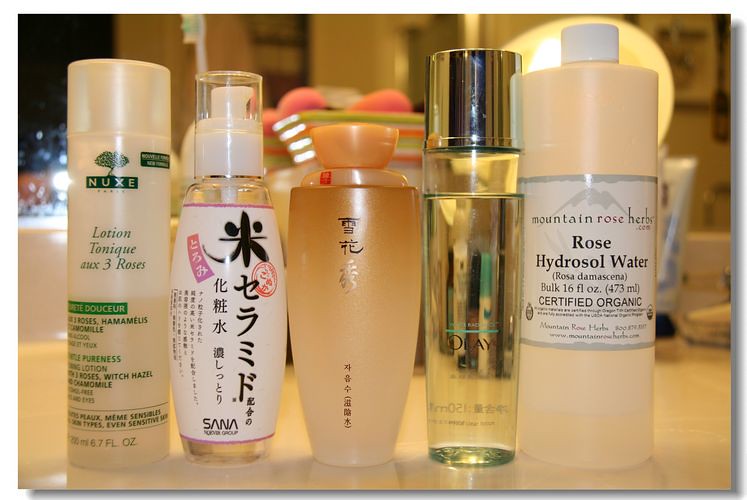In this image, a collection of various beauty and wellness products is displayed, each with distinctive packaging and brands. On the far left, there is a Nuxe product, a renowned French brand known for its luxurious skincare. This particular item appears to be a lotion or tonic, packaged in a 6.7 fluid ounce bottle with a design that features illustrations of roses, witch hazel, and chamomile, likely denoting its soothing and herbal qualities.

Next to it is a small container, possibly a body spray or body oil, characterized by its unique shape—wider in the middle and tapering towards the top. The container is fitted with a pump mechanism, secured by a clear plastic lid. Its label is adorned with numerous Asian characters, indicating it might be a product of either Chinese or Japanese origin, though the specific details are not readable.

The central item could be identified as a perfume or lotion, housed in a frosted container with an opaque, clear finish. Like the aforementioned product, it also features foreign characters on the label, suggesting its international source.

Following this, there is a clear bottle that appears to be a fragrance product from Olay, a well-known brand in skincare and beauty products. The simple yet elegant design of the bottle hints at a minimalist aesthetic, focusing on clarity and purity.

The final item is an essential oil from Mountain Rose Herbs, packaged in a utilitarian container commonly used for larger volumes of essential oils. This one is labeled as Rose Hydrosol Water, a 16 fluid ounce bottle that is certified organic. The packaging is functional with a frosted clear glass that allows visibility of the liquid level inside.

This curated collection showcases a variety of skincare and wellness products, ranging from luxurious lotions to functional essential oils, each with distinct branding and origins.